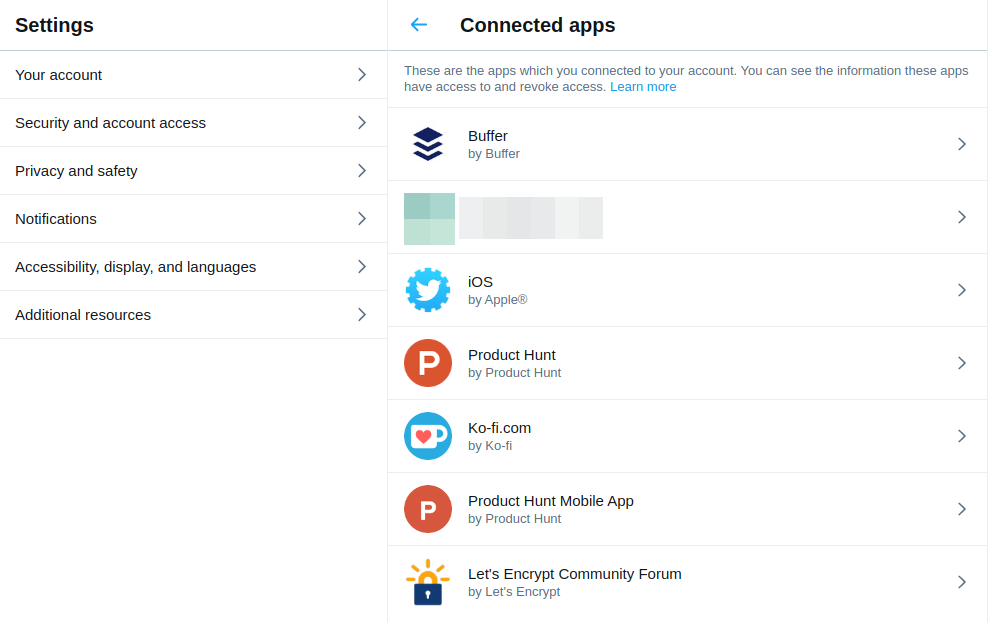The image is a screenshot of a user interface, specifically from a settings page where connected applications are managed. The layout features a two-column design. On the left side, there is a vertical navigation panel with multiple tabs, each labeled: 

- Settings
- Your Account
- Security and Account Access
- Privacy and Safety
- Notifications
- Accessibility, Display, and Languages
- Additional Resources 

The primary area on the right side displays the content for the "Connected Apps" tab. This section is headed by the title "Connected Apps," accompanied by a blue arrow icon. Below the title, there is informational text explaining that these are the applications connected to the user's account, detailing that you can view the information these apps have access to and revoke access if needed. Additionally, there is a "Learn More" link in blue font for further information.

Below this explanatory text, the connected applications are listed. The first app in the list is "Buffer by Buffer." The second app's name and details are obscured in the screenshot. The subsequent apps are listed as follows:

- iOS by Apple
- Project Hunt by Product Hunt
- Coffee.com by Coffee or CoFi
- Product Hunt Mobile App by Product Hunt
- Let's Encrypt Community Forum by Let's Encrypt